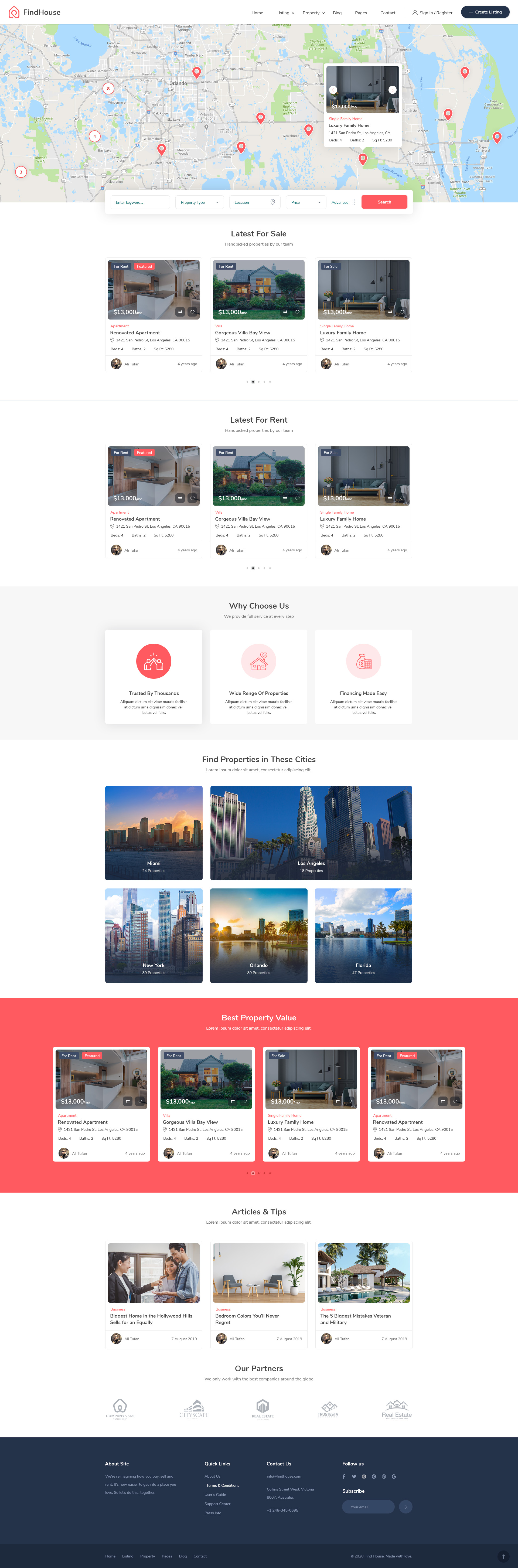This image showcases a comprehensive view of a real estate website, displaying the entire webpage in a single screenshot. In the top left corner, the site features the text "Find House" alongside a small red house icon encircled by a design element. The header also includes multiple tabs and a prominent blue button.

Moving down, the website highlights an interactive map in a grayscale theme, illustrating various roads and marked by red icons. There is a pop-up overlay providing a preview of a property interior.

Below the map section, the site categorizes listings with headings such as "The Latest For Sale," showcasing three property thumbnails—two of interiors and one of an exterior. Following this, "Latest For Rent" is displayed, featuring the same set of images.

Further down, the site promotes its strengths with a section titled "Why Choose Us," illustrated by several white boxes containing icons. 

Next, a gallery of six images of different outdoor settings accompanies the heading "Find Properties in These Cities." Following this, a highlighted section in red titled "Best Property Value" appears, displaying multiple property thumbnails.

Towards the bottom, a section named "Articles and Tips" includes additional thumbnails, providing further resources for site visitors.